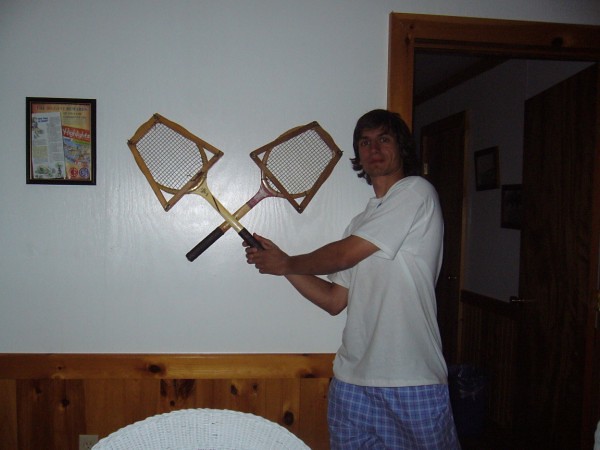The photograph captures an older image of a man standing in a room beside a doorway that leads to a dimly lit hallway with dark wooden doors and doorframes. The man, who has slightly longer hair, is wearing a white shirt paired with blue and white checkered shorts. He is holding two tan wooden tennis rackets with black handles—one in each hand, creating a crossed effect, as they appear to be mounted on the wall. The racks and his grasp give the impression that he is holding them. The wall behind him is white on top with wooden paneling below, approximately waist-high. Alongside the rackets on the wall, there is a framed picture that looks like a magazine piece, and another set of framed newspaper clippings, although the content is indiscernible due to the image quality. Additionally, at the very bottom of the image, there is a semi-oval object that might be a piece of furniture or fabric, like a chair or sweater, but its exact nature is unclear. The photograph gives a nostalgic feel, reminiscent of older digital cameras or early mobile phones.